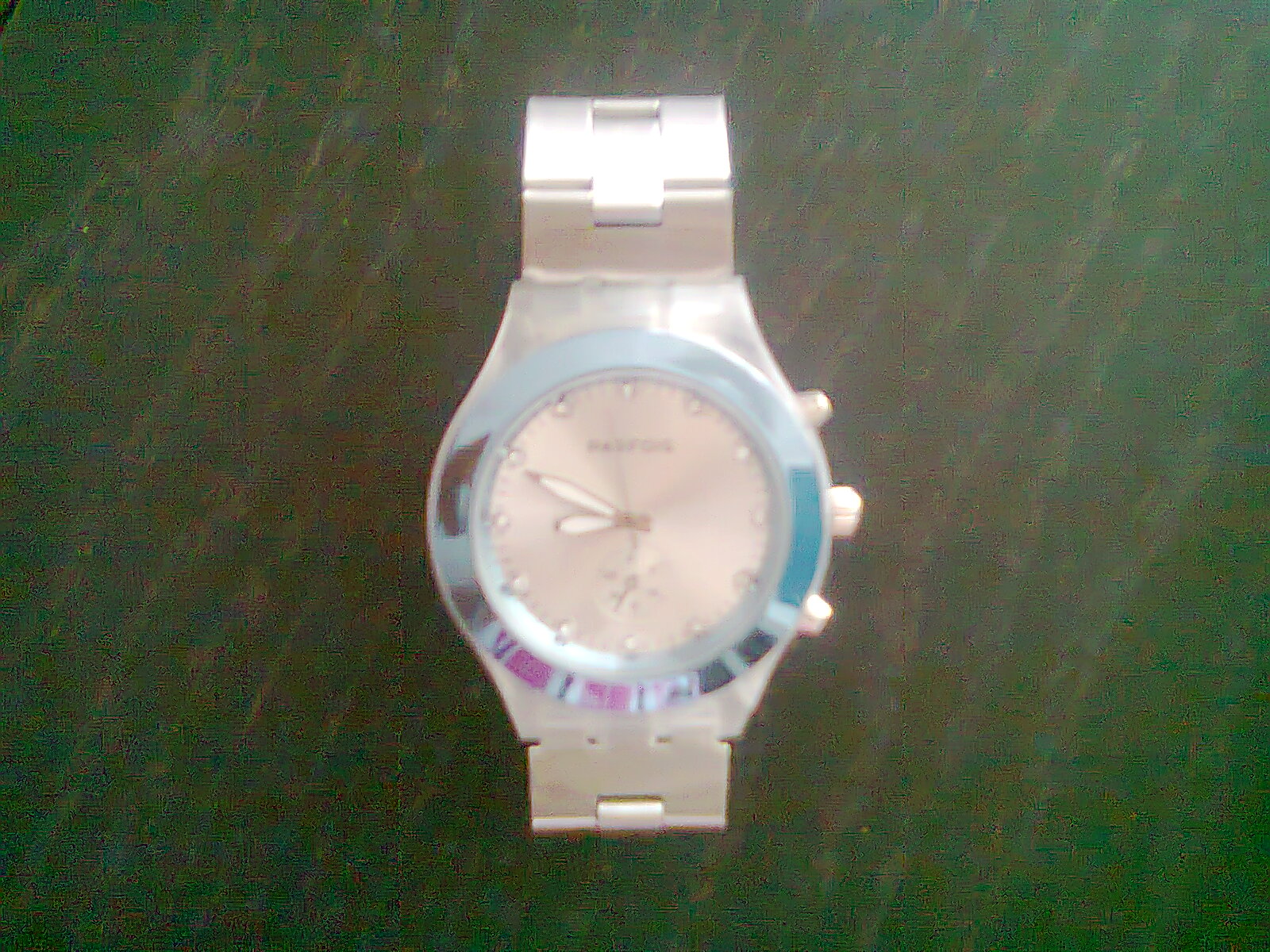A blurry and grainy photograph captures a silver watch resting on a textured green surface, possibly painted wood. The watch features a linked silver band and a white face with rounded hour and minute hands indicating the time as approximately 8:49 or 8:50. Surrounding the watch face is a bluish-silver bezel, which may be reflecting ambient light, adding a purplish hue at the bottom. The watch includes three functional dials on its right side: a central, thicker winding dial flanked by buttons positioned above and below it along the curve of the watch. The overall image quality is poor, appearing washed out due to excessive lighting.